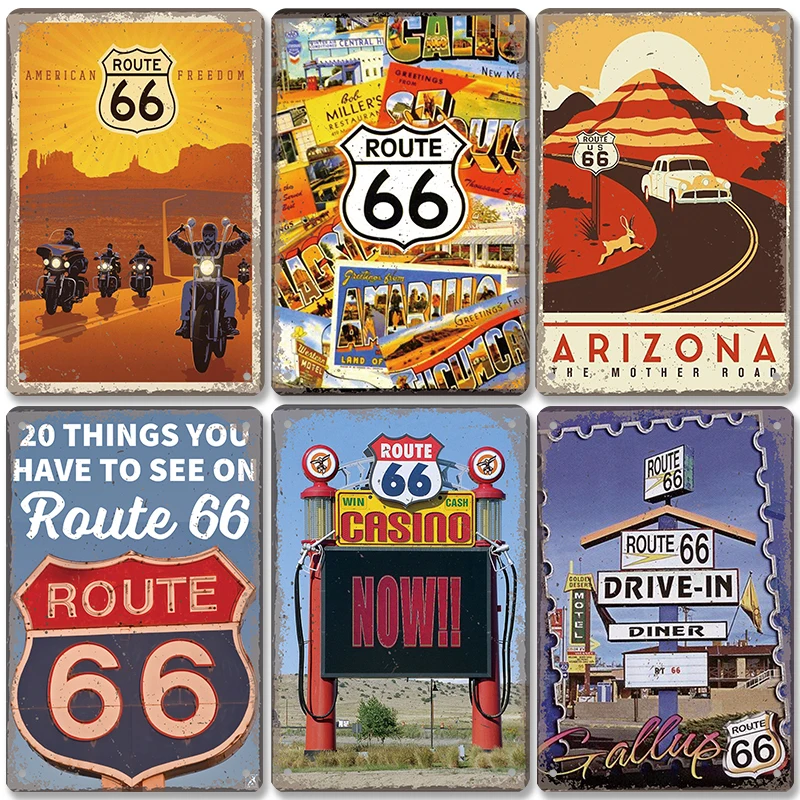This image showcases six distinct, rustic metal signs, all themed around the iconic Route 66 highway, famous for traversing through the American West. Arranged in a grid of three on the top and three on the bottom, each sign vividly captures different aspects of the Route 66 experience in a variety of bright, desert-inspired colors like rust, gold, red, orange, blue, and yellow.

Starting from the top left, the first sign features an illustration of motorcycle riders journeying through the iconic Monument Valley, accompanied by the phrases "American Freedom" and "Route 66." The top center sign presents a collage reminiscent of old-fashioned postcards, adorned with vivid colors and mentioning "Bob Miller, New Mexico." The top right sign illustrates a car driving along a desert highway in Arizona, with a rabbit leaping across the road and the words "Route 66" prominently displayed.

On the bottom left, a simple yet informative sign highlights "20 things you have to see on Route 66." The bottom center sign, styled like a gas pump, advertises the "Gwynn Cash Casino Now" along the Route 66 path. Finally, the bottom right sign is a playful combination sign for a "Route 66 Drive-in Diner" and a motel, evoking the nostalgic feel of a roadside stop.

The detailed diversity in imagery and text across these signs collectively captures the cultural and historical essence of Route 66, offering a vibrant and eclectic visual journey.